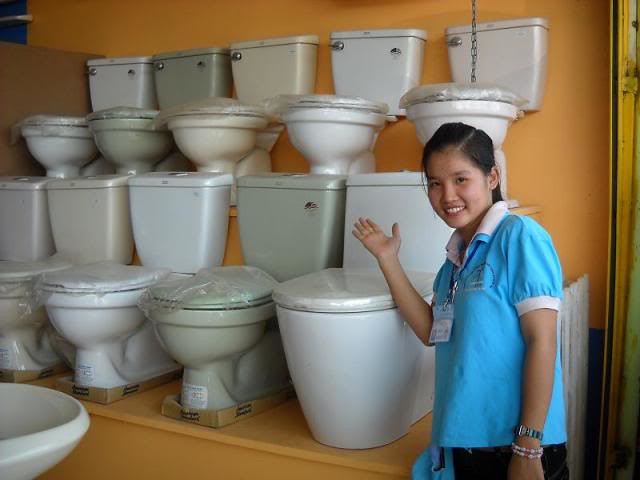The image captures an Asian woman, likely a sales associate at a store, posing next to a display of new porcelain toilets. She is standing to the right of the display, smiling at the camera with her right hand stretched out, palm open, gesturing towards the toilets. The woman has black hair pulled back and is wearing a blue shirt with puffed, short sleeves, each trimmed in white, along with a white-collared lanyard around her neck holding her ID tag. She also sports a watch and two bracelets on her left wrist. The display features ten toilets in total, with five on an upper orange shelf and five on a lower matching shelf. The toilets come in various colors, including white, light green, and cream, with their seats wrapped in plastic. The background features an orange wall, and there is a porcelain sink partially visible across from the shelves.